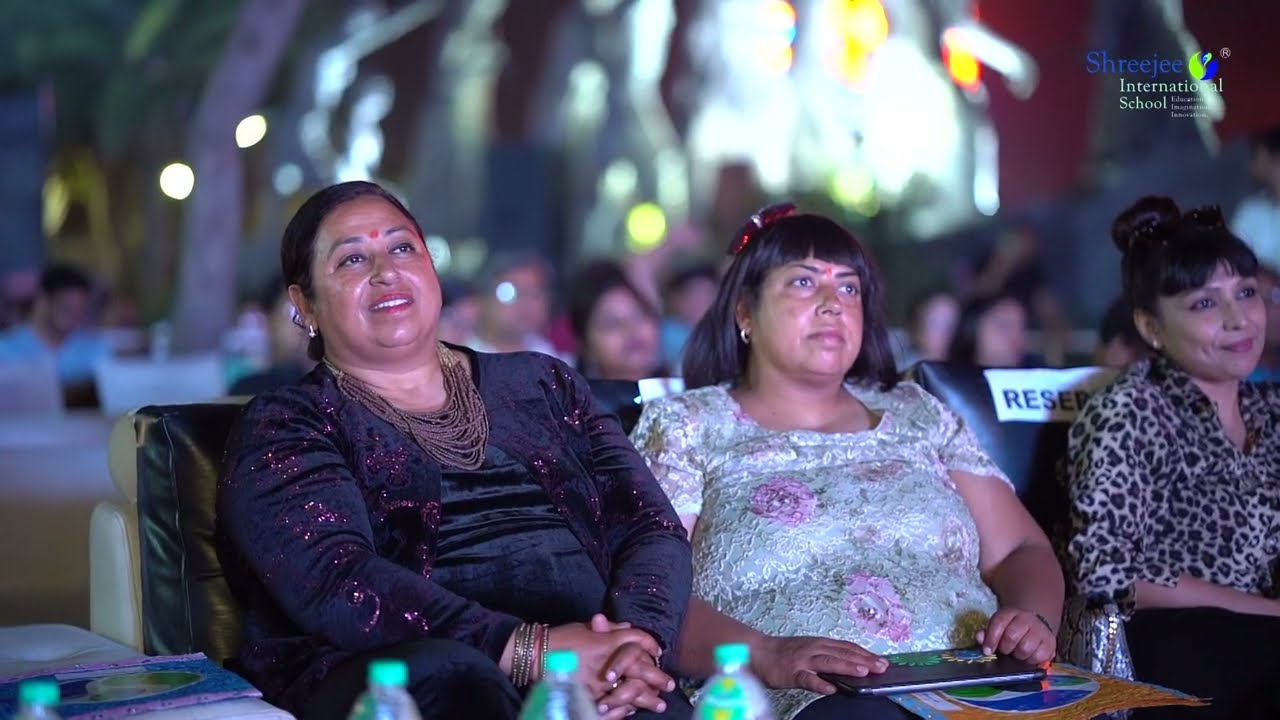In this horizontal and rectangular image, a group of Indian or Pakistani women is seated in a theater, possibly watching a movie or attending a performance. The three primary women featured prominently in the foreground all have dark brown or black hair and red dots on their foreheads. The woman on the left is dressed in a black dress adorned with multiple necklaces, with her hair tied back. The central woman, slightly overweight, wears a white dress with pink flowers and a red bow in her hair. To the right, the third woman has her hair in a bun and wears a leopard-print black and beige top with black pants. They are all seated in black leather seats, and the back of one chair is marked "reserved." Behind them, blurred figures indicate more people also seated and looking up at an unseen screen or stage. The tops of clear plastic drink bottles with light green lids line the bottom of the picture horizontally. In the upper right corner, some text is visible in blue, yellow, and green, though it is not fully legible.